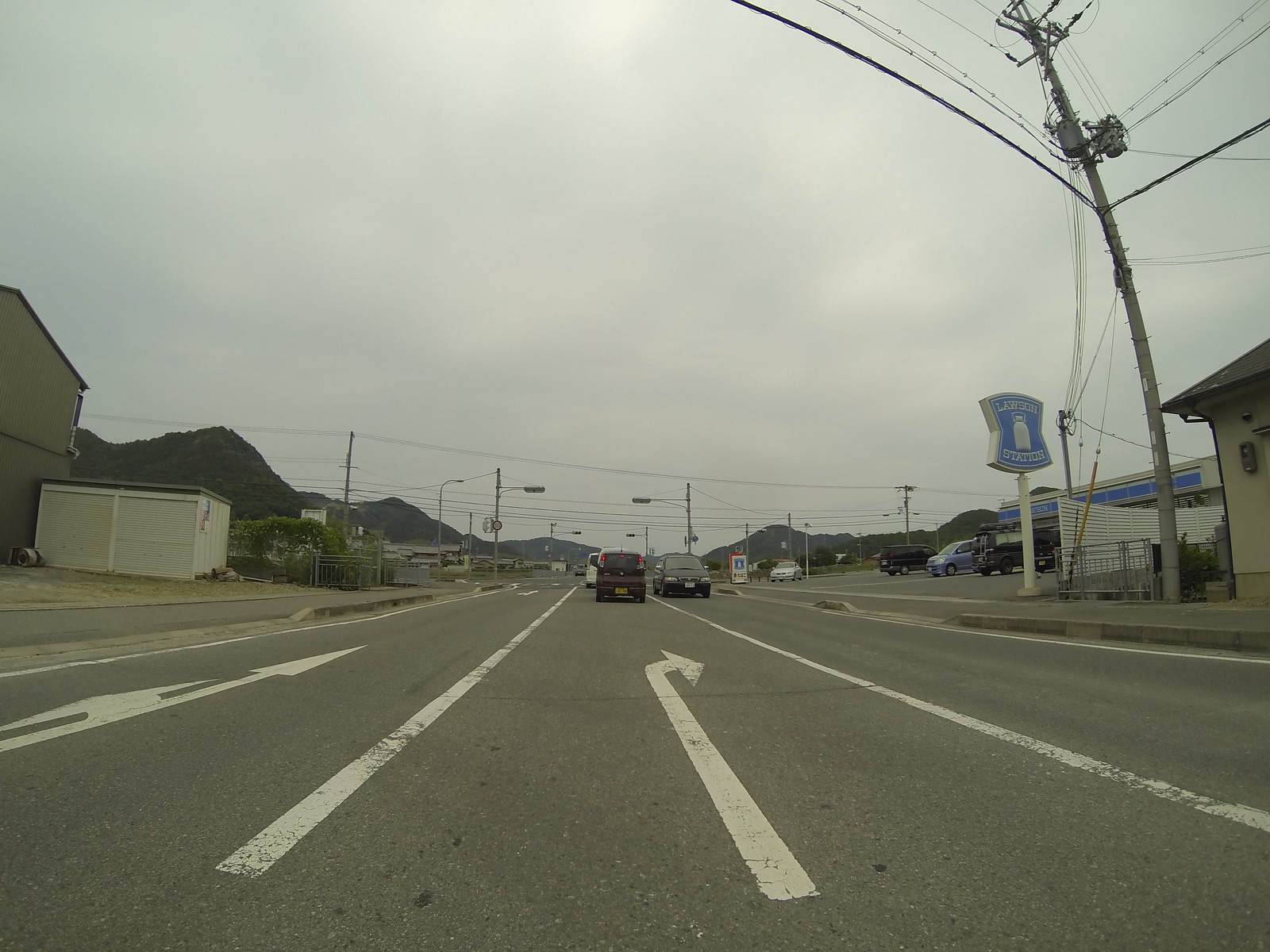The image captures a bustling urban street from a downward angle, revealing a scene layered with various elements. On the right side, a towering power pole stands prominently near the road, its angle distorted by the lens, giving it a seemingly bent and rounded appearance. Adjacent to the pole, the edge of a residential house marks the beginning of the frame. A distinct white sign with a blue top stands out nearby, possibly indicating a business or traffic information. The street itself is lined with several cars parked along both sides, indicating active businesses and heavy foot traffic. The road splits into three lanes: one designated for regular traffic, another for drivers intending to turn right, and a third for those going straight or turning left. On the left side, a white garage is visible, hinting at the end of an apartment complex. The scene is alive with quite a bit of traffic, featuring numerous vehicles moving or parked, contributing to the lively atmosphere of the thoroughfare.